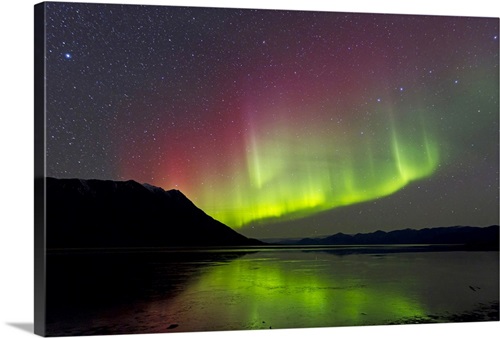This image is a high-resolution nighttime photo of the Northern Lights, beautifully showcasing the aurora borealis over a serene, icy landscape. The photograph, printed on a canvas and wrapped around the edges of a box frame, captures the ethereal beauty of the lights as they cast an entrancing glow across a tranquil, frozen bay flanked by towering mountains. The bay's smooth, ice-covered surface mirrors the dazzling lights above, creating a hauntingly beautiful effect. The aurora displays traditional vertical streaks in hues transitioning from vibrant green at the bottom through goldish highlights to rich purple-red at the top. Behind the shimmering lights, the night sky is punctuated by a multitude of small, white stars, including one particularly bright star on the left. This intricate photo, possibly taken in northern Canada, also subtly features floating materials along the shoreline, potentially vegetation mingled with ice, adding to the natural allure of the scene. The entire composition, shadowed against a dim background, creates a mesmerizing, luminous spectacle that is at once haunting and beautiful.